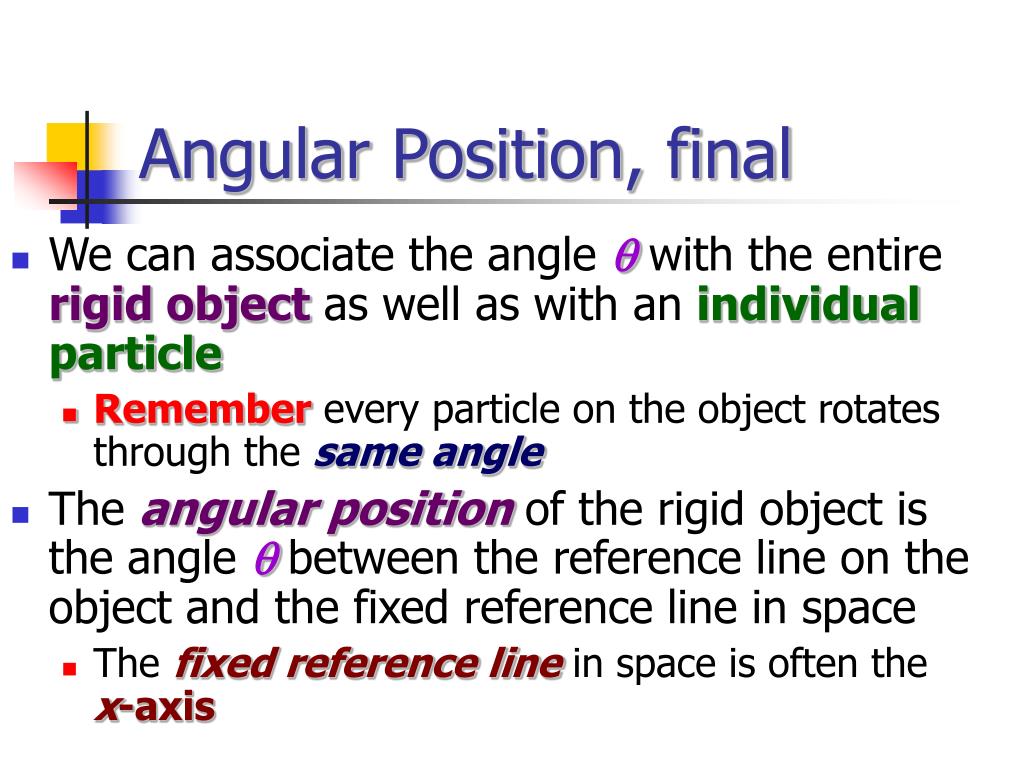The image resembles a PowerPoint slide, prominently featuring textual information and a particular color-coded design. In the upper left corner, three overlapping gradient squares in yellow, red, and blue are connected by thin black lines that form a simple yet structured design. To the right of these squares, the phrase "angular position, final" is displayed in blue font. Below, several bullet points detail important concepts.

The first bullet point, marked with a blue square, states: "We can associate the angle θ with the entire rigid object as well as with an individual particle." Here, "θ" appears in purple, and "individual particle" is in green.

Following this, a red bullet point reads: "Remember, every particle on the object rotates through the same angle," with "Remember" in red and "same angle" in blue.

Another blue bullet point explains: "The angular position of the rigid object is the angle θ between the reference line on the object and the fixed reference line in space." The terms "angular position" and "θ" are highlighted in purple.

Concluding, a red bullet point states: "The fixed reference line in space is often the x-axis," with "fixed reference line" and "x-axis" appearing in a darker red or burgundy color. The entire slide is structured as an instructional text, possibly for a lecture or presentation on angular positions in physics.